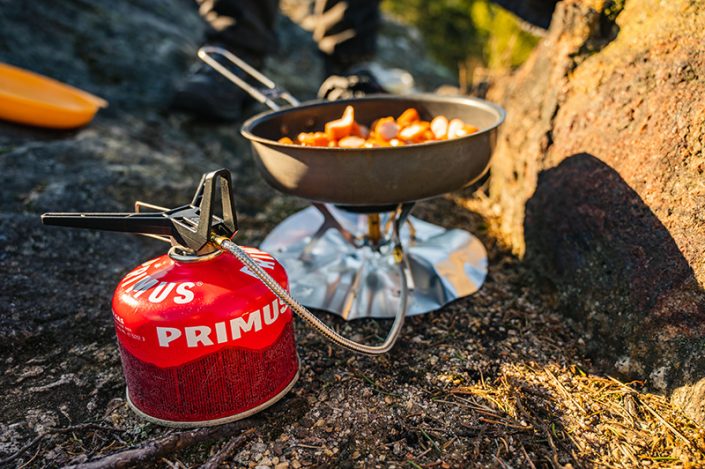The image depicts an outdoor cooking scene in a rugged, uneven dirt area scattered with rocks. Central to the image is a gray metallic pan with a handle positioned to the upper left, containing chopped food with white, orange, and yellow chunks, possibly meat. The pan rests on a metallic, crumpled circular base, part of a small gas burner setup. The burner connects via a hose to a short, squat, red gas canister emblazoned with "Primus" in bold white letters. The gas tank sits to the left of the burner, with a tube extending from its black connector. In the background, there are some blurry rocks and patches of grass, while the bottom right corner features some brown grass. There is also an indistinct yellow plate visible in the upper left corner. A large rock protrudes into the image from the right side, contributing to the rugged outdoor ambiance.